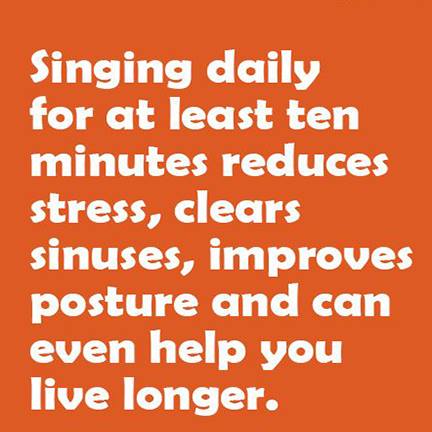The image consists of a motivational text set against a vivid orange background. The bold white letters of the text read, "Singing daily for at least 10 minutes reduces stress, clears sinuses, improves posture, and can even help you live longer." The sentence begins with a capitalized 'S' and spans eight lines, taking up the majority of the image. The simple, playful design and vibrant color scheme give it a lighthearted feel, making it suitable for sharing on social media platforms like Instagram or Facebook. Despite the slight blurriness, the message remains clear and uplifting.